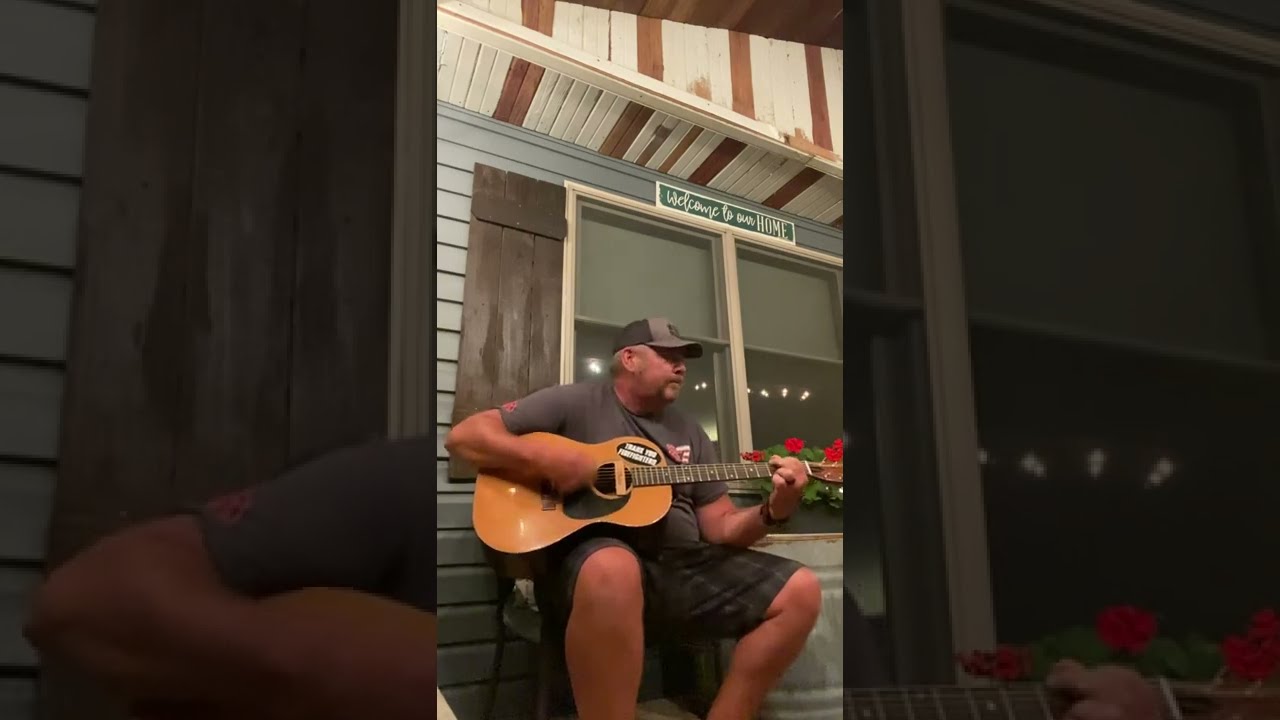In the center of the image, we see a man sitting and playing a brown acoustic guitar with a black sticker that might read "Thank you firefighters" in white text. He is wearing a gray t-shirt, dark gray plaid shorts, and a gray and black baseball hat. The man is seated in a wooden chair with wooden legs and a white seat. 

The background features a blue building with white-framed windows and black shutters. Above the window behind the man, there's a green sign with white text that reads "Welcome to our home." To the right side of the window, a basket hangs filled with red roses, adding a touch of color to the scene. 

The image is flanked on both sides by zoomed-in portions of the central image, enhancing the focus on details of the man and his guitar. It is a bright and relaxed setting, suggesting he is either outside or in a well-decorated porch area.